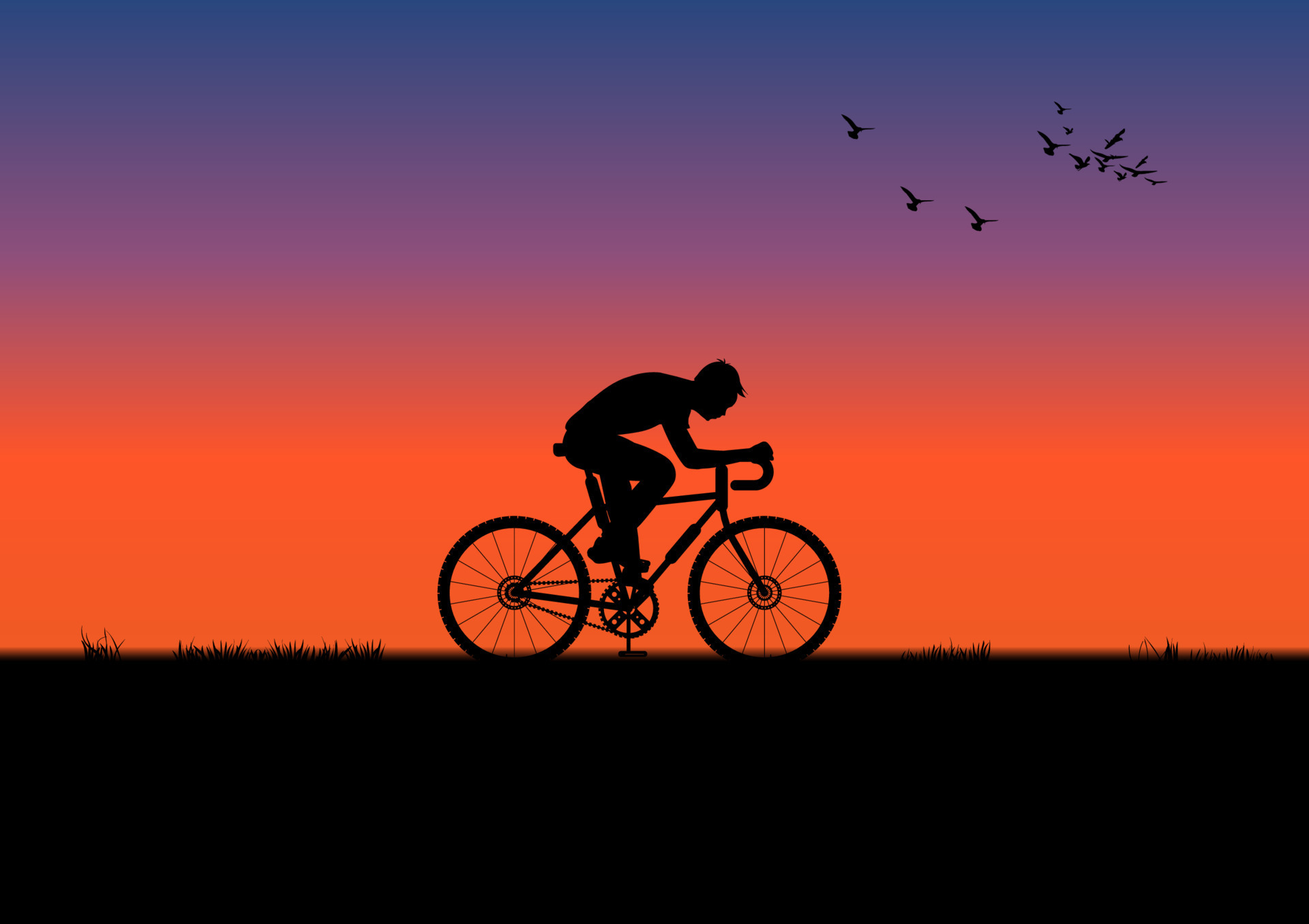The image showcases a stunning piece of digital artwork, depicting an evocative twilight scene. The sky transitions from a reddish-orange glow at the center to a strip of luminescent purple above, and finally a deep blue at the top third. Against this vivid backdrop, a flock of about a dozen black birds flies in the upper right-hand corner, within the blue and purple zones of the sky. Below, the dark foreground appears to be a park or pathway, punctuated by sporadic blades of grass. Silhouetted by the glowing horizon is a bicyclist riding a two-wheeled bike. The rider, leaning forward onto curved handlebars, wears a possible ball cap, creating a dynamic and captivating silhouette against the majestic, colorful sky.